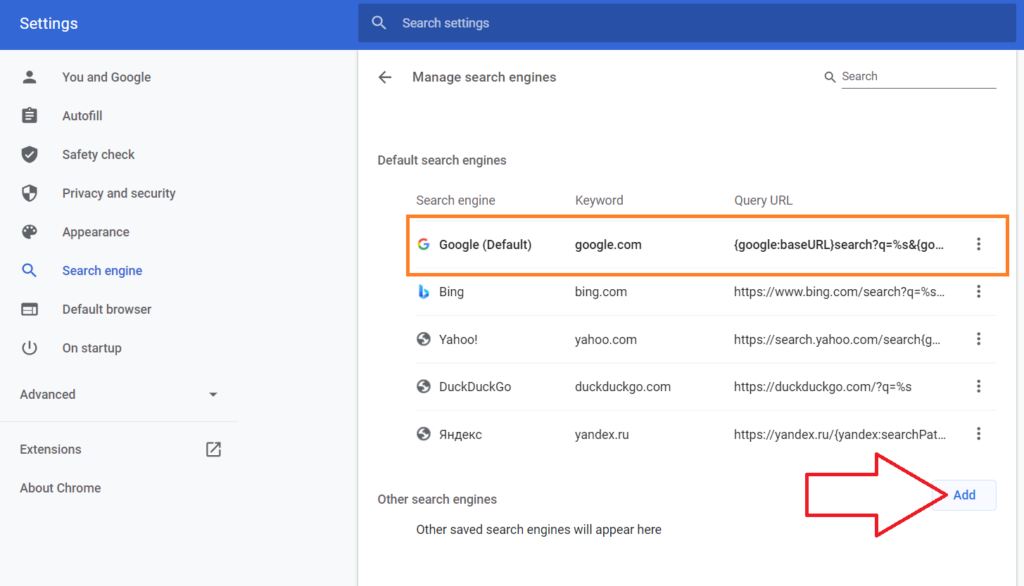The image depicts a settings menu, likely from a Windows environment, with a layout that is approximately 50% wider than its height. The upper 10% of the menu features a horizontal blue header. On the left side of the header, gray text reads "Settings," and about 40% to the right of this text is a search bar. This search bar has a darker blue background with a gray magnifying glass icon and the text "Search Settings" within it. 

A vertical divider line splits the upper section, placing the search bar on the right. Below this, on the left, a vertical menu lists various settings categories, each accompanied by an icon. The categories are:

1. You and Google
2. Autofill
3. Safety Check
4. Privacy and Security
5. Appearance
6. Search Engine (highlighted in blue, indicating it is the current selection)
7. Default Browser
8. On Startup

Below these options, a drop-down menu labeled "Advanced" can be extended, followed by options for "Extensions" and "About Chrome."

The right-hand section of the image displays the  "Search Engine" settings, indicating that the current focus is on managing default search engines. Additional options and settings related to search engines are visible below this heading.